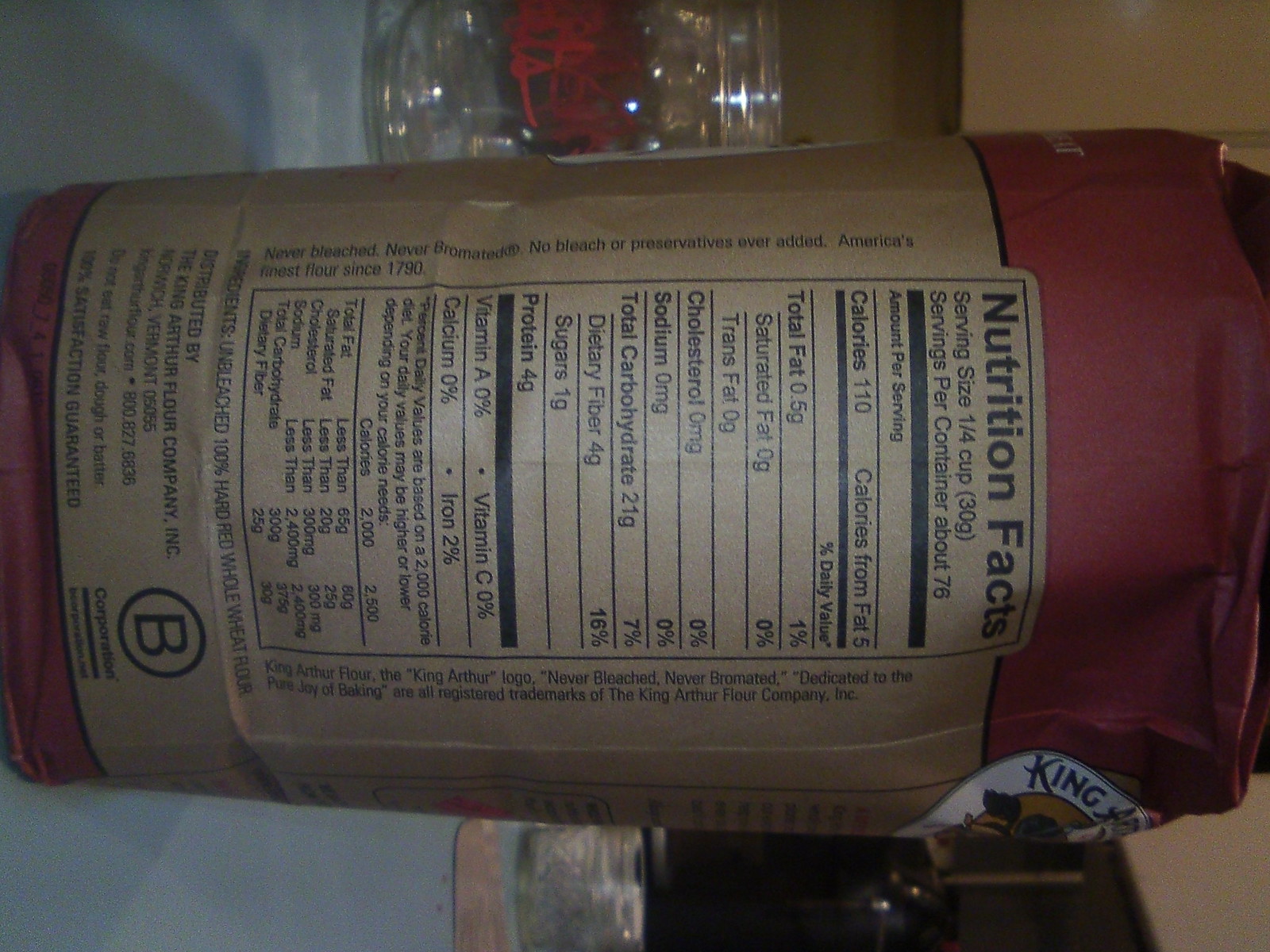The image captures a first-person perspective of the nutrition facts label on a food packet. To read the nutritional information correctly, you'd need to tilt your head 90 degrees to the right, as the image has been rotated similarly. The packet appears to be made of paper, featuring a distinctive color scheme with a brown middle section flanked by smaller red sections on the top and bottom. 

The nutrition table provides the following information:
- **Serving Size:** 1/4 cup (30 grams)
- **Servings Per Container:** About 76
- **Amount Per Serving:**
  - **Calories:** 110
  - **Calories from Fat:** 5
- **Nutritional Breakdown:**
  - **Total Fat:** 0.5 grams (1% Daily Value)
  - **Saturated Fat:** 0 grams (0% Daily Value)
  - **Trans Fat:** 0 grams
  - **Cholesterol:** 0 milligrams (0% Daily Value)
  - **Sodium:** 0 milligrams (0% Daily Value)
  - **Total Carbohydrates:** 21 grams (7% Daily Value)
  - **Dietary Fiber:** 4 grams (16% Daily Value)
  - **Sugars:** 1 gram (No Daily Value listed)
  - **Protein:** 4 grams (No Daily Value listed)
- A black bar separates the main nutritional information from vitamin details:
  - **Vitamin A:** 0%
  - **Vitamin C:** 0%
  - **Calcium:** 0%
  - **Iron:** 2%

Additionally, a note at the bottom of the table mentions that these percentage daily values are based on a 2,000-calorie diet, and daily values may be higher or lower depending on individual calorie needs.